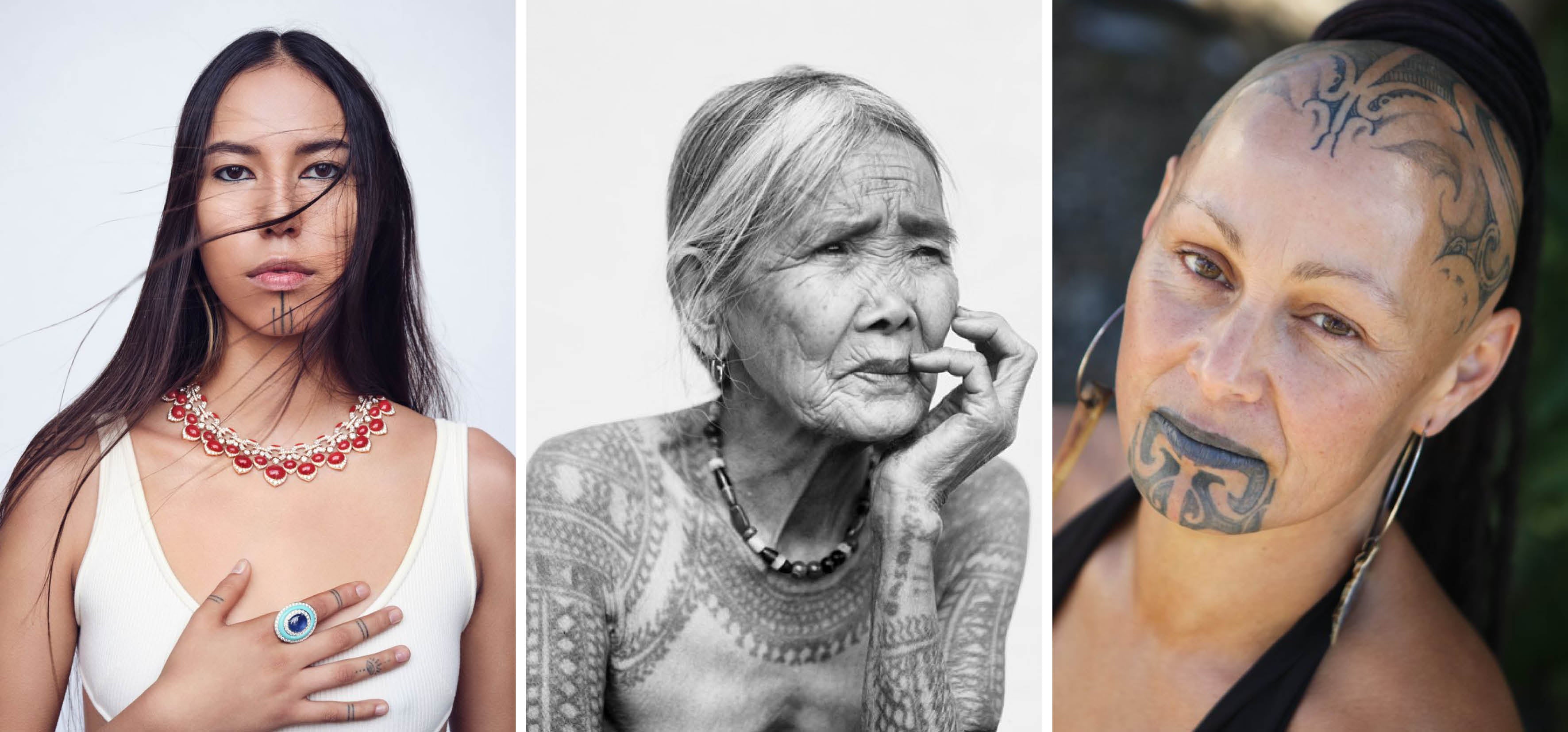The image is a horizontal triptych of photographs showcasing three Native American women. The leftmost portrait is a vertical color image of a young woman in her early 20s. She has long, straight black hair cascading past her shoulders, and black eyes framed by black eyebrows. She wears a detailed, silver-tone necklace adorned with red beads and stones. She's dressed in a white tank top, and her right hand, adorned with a turquoise and black opal ring on her index finger, is crossed over her chest. In the center is a striking black-and-white photograph of an elderly Native American woman. Her face is lined with wrinkles, and her hair is straight and pulled back. She wears a beaded necklace and has extensive tattoos covering her arms, shoulders, and neck. The woman's gaze is directed off-camera, suggesting contemplation. The rightmost image features a bald Native American woman with tattoos on her chin and scalp. She wears large hoop earrings and a black tank top. Her lips appear to be darkened with tattoos, and she is gazing directly into the camera. All three women, each bearing unique tribal tattoos and jewelry, reflect their cultural heritage with solemn and reflective expressions.